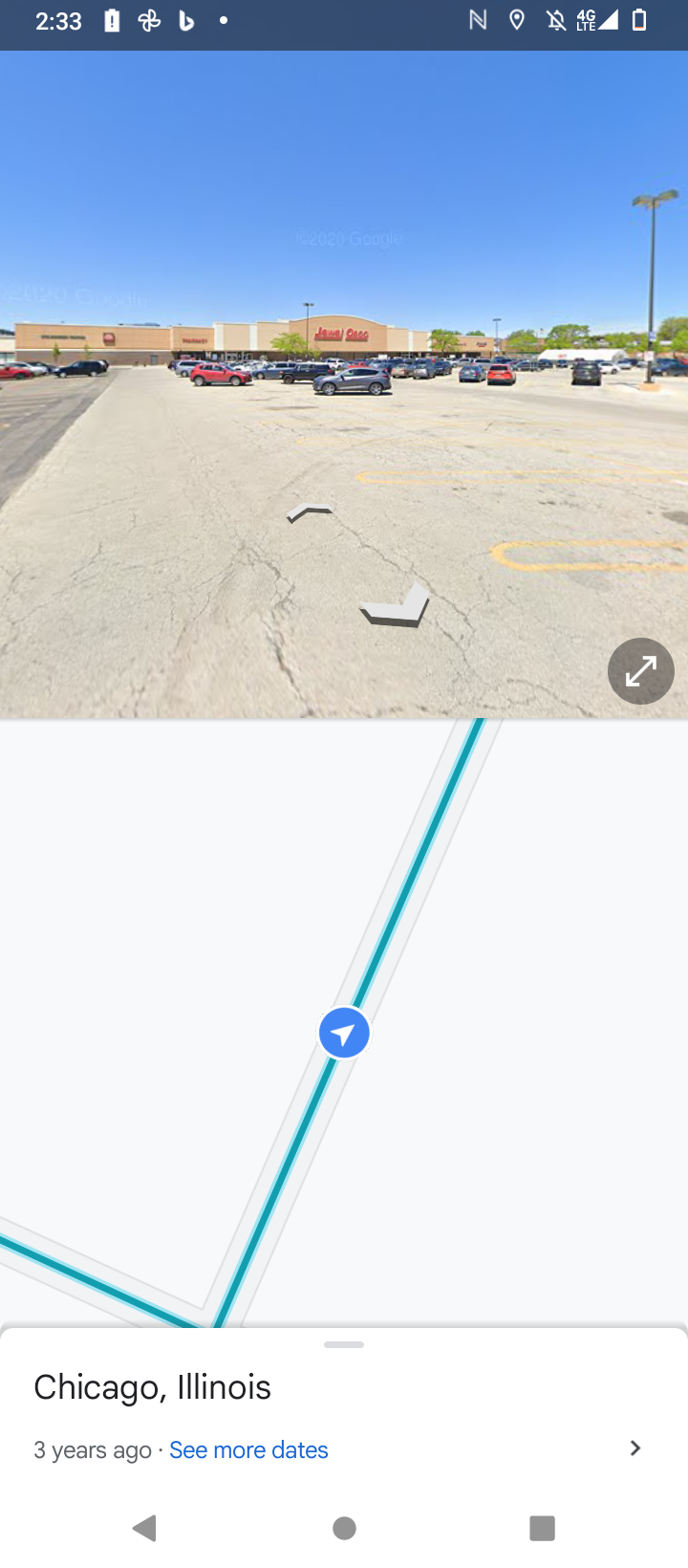A detailed screenshot from a phone screen captures a bustling parking lot adjacent to a large chain store. Occupying the top part of the image is the store's name, though partially obscured. The parking lot itself is nearly full, indicating a busy day. Below this, a map icon is prominently featured, marking a specific location. A blue arrow points to "Chicago, Illinois," alongside a timestamp reading "three years ago," with an option to "see more dates" available. Along the top of the screen, typical smartphone indicators are displayed, showing the time as 2:33, along with battery life and network connectivity status, providing a glimpse into the phone's interface and context.